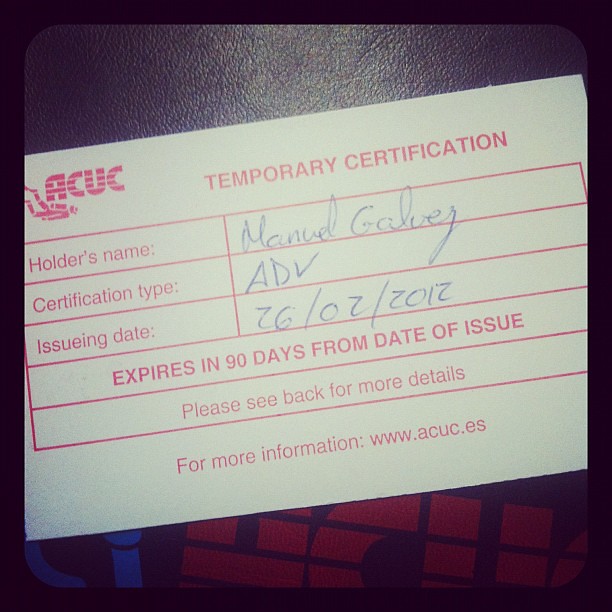In the image, we see a close-up photograph of a temporary certification card resting on what appears to be a black leather couch. The white card prominently features red and blue text. In the upper left corner, the red and white logo "ACUC" is displayed, followed by the red text "Temporary Certification" at the top center. The card includes several labeled sections: "Holder's Name," "Certificate Type," and "Issuing Date," with the respective details filled in blue pen: "Manuel Galvee" as the holder's name, "ADV" as the certificate type, and "26-02-2012" as the issuing date. Below these details, in red text, it states "Expires in 90 days from date of issue." At the bottom of the card, instructions read "See back for more information" and "For more information www.acuc.es." The card is bordered by the black leather background, with some additional object featuring black with blue and red lettering partly visible underneath.